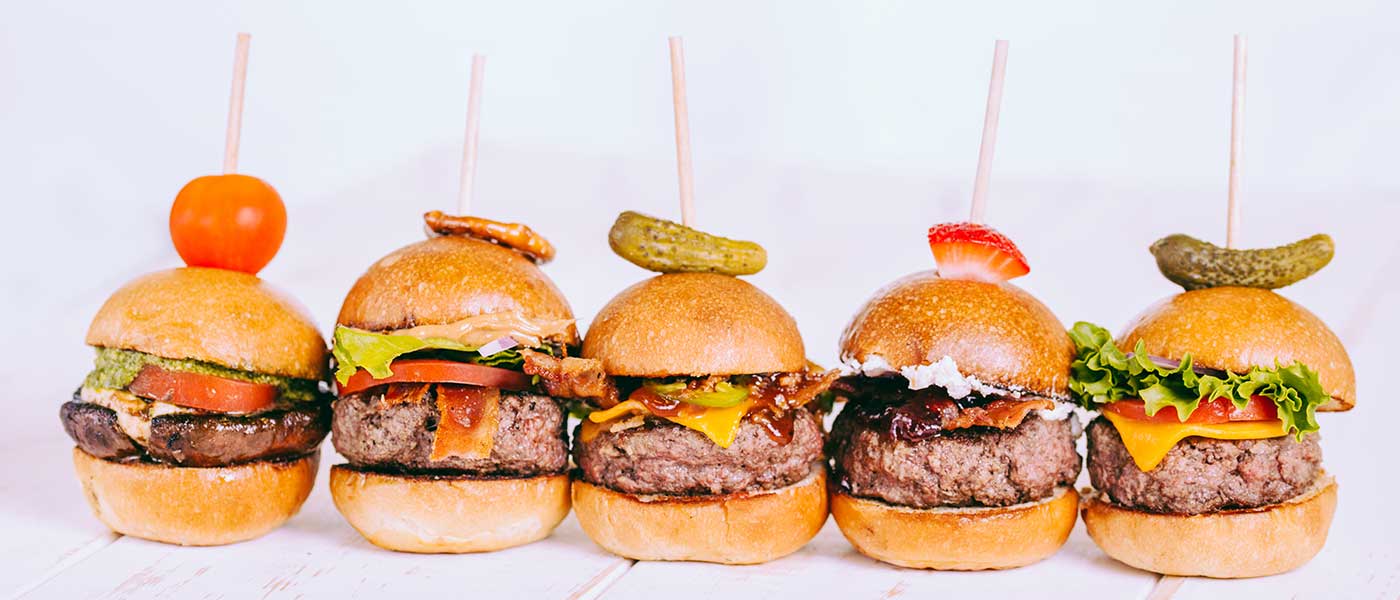This vibrant photograph showcases five miniature cheeseburgers, perfectly aligned from left to right against a pristine white background. Each slider features a golden-brown bun, a juicy beef patty, and standard toppings of fresh lettuce and tomato. The toppings, however, greature unique variations: some burgers sport a slice of creamy white cheese, while one includes crispy bacon for added flavor. To add an artistic touch and ensure stability, each burger is skewered with a stick adorned with different items: a cherry tomato, a gherkin pickle, a piece of strawberry, and a pretzel. This arrangement not only prevents the sliders from toppling but also creates a visually appealing and colorful presentation.